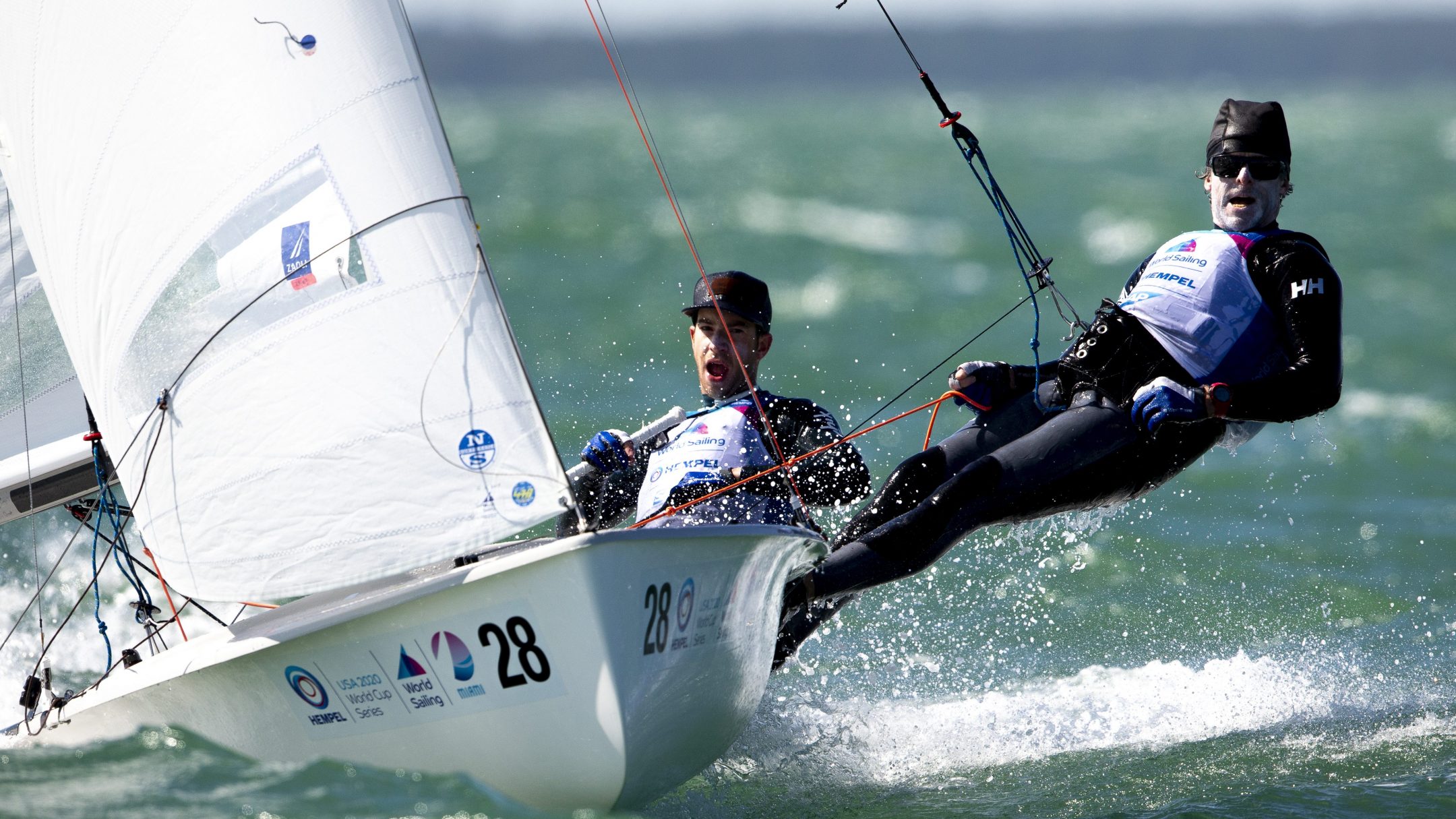In the photograph, a sleek white sailboat races through greenish ocean waters with two professional sailors expertly maneuvering it. Both sailors, dressed in black wetsuits and matching black caps, are distinctly positioned on the right side of the boat. The man at the rear is intently focused on controlling the rudder, while the other is dramatically leaning back, almost parallel to the water, as he manages an orange rope tied securely to the boat's mast via a black belt adorned with brass holes. Emphasizing its competitive nature, the sailboat proudly displays the number "28" on both sides along with several distinctive stickers and logos. Notable among these are “Hemphill” in a blue circle, "USA," "World Cup Series," "World Sailing," and “Miami.” The sailors’ bibs and the meticulous details on the boat suggest that this is a high-level competition, possibly the 2020 World Sailing Cup in Miami. The blurred background adds to the sense of speed and focus required for this intense sailing endeavor.